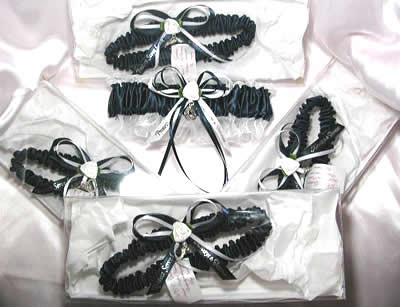This is a detailed black and white photograph showcasing a collection of five garter belts or elastic wristbands, each adorned with black and white striped bows. The garters are composed of a thick, stretchy material designed to fit various sizes, and they feature a central medallion or embellishment, possibly heart-shaped. Each garter is presented in its own rectangular box lined with a white, silky fabric. The central focus is a garter displayed horizontally in a foreground box with a bow tied in front, accompanied by a small tag in the lower left. Behind this, two garters are arranged diagonally in their boxes, pointing towards the upper corners of the image. Another garter is centered in the upper portion, and one more is situated at the top, all set against what appears to be an off-white silk sheet. No text or printing is visible in the image.